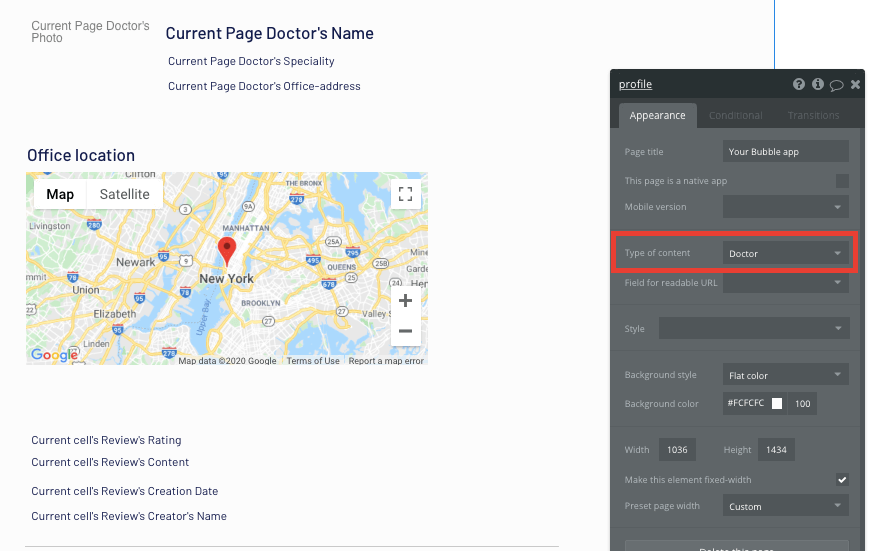This image showcases a setup for a Google business page tailored for a doctor's office. On the left side of the image, there is a prominent, large white box resembling a template for a doctor's Google business search page. At the top left corner of this box, there is a placeholder labeled "Current Page Doctor's Photo," indicating where the doctor’s photo would be placed. To the right of the placeholder, the text "Current Page Doctor's Name" is displayed in bold blue letters. 

Below that, in smaller blue letters, the text lists the "Current Page Doctor's Specialty," "Current Page Doctor's Office Address," and central to the template, the words "Office Location" are prominently displayed. Beneath this heading on the left, there is a rectangular map image with a pin drop in the center, showing that once the office address is updated, the pin will adjust accordingly on the map. At the bottom left corner of the template, there's information regarding contact details such as a cell phone number, user reviews, and additional relevant information.

To the right of the page, there is an overlay of a mobile phone screenshot illustrating editing tools for the web page. These tools include options like "Page Title," whether the page is a "Native App," "Mobile Version," and the "Type of Content." This section is highlighted with a red box indicating that "Doctor" is selected as the content type.